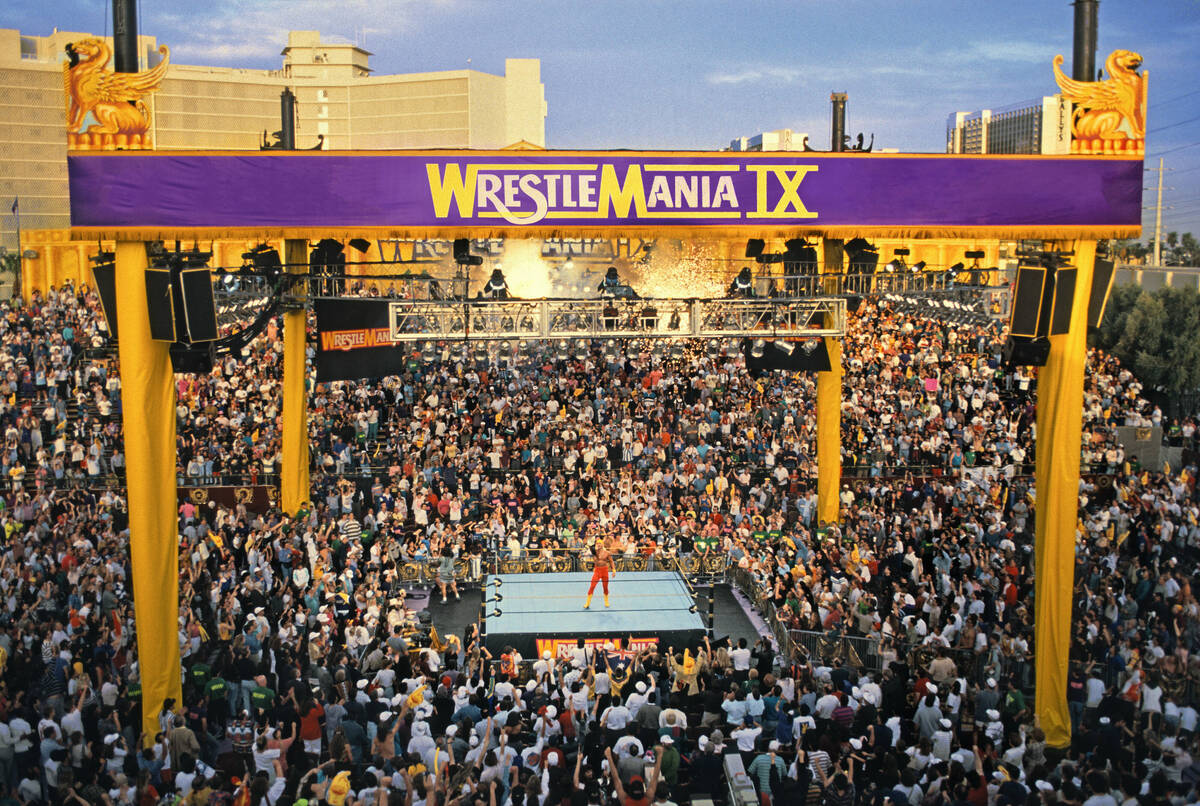This dynamic outdoor photograph showcases the grand spectacle of WrestleMania IX, set against a medium blue sky speckled with white clouds. The focal point is the centrally located wrestling ring, appearing small due to the high vantage point of the camera. The ring is surrounded by a vast, enthusiastic crowd filling both the base area and the adjacent stands. Towering above the scene are four large tall yellow-covered poles, supporting a grand structure that includes various speakers and lighting equipment. Prominently displayed in the center of this structure is a striking purple banner with the bold yellow letters "WrestleMania IX," where the acronym "WM" and the numeral "IX" are in bright yellow, and the letters "R-E-S-T-L-E-M-A-N-I-A" are in a lighter yellow. In the middle of the ring stands a wrestler, proudly holding a championship belt over his right shoulder. He is dressed in red pants and yellow boots, adding a vivid splash of color to the scene. The photograph captures the vibrant atmosphere of the event, enhanced by the urban backdrop of city buildings, suggesting the possibility that this spectacle might be set in Las Vegas.